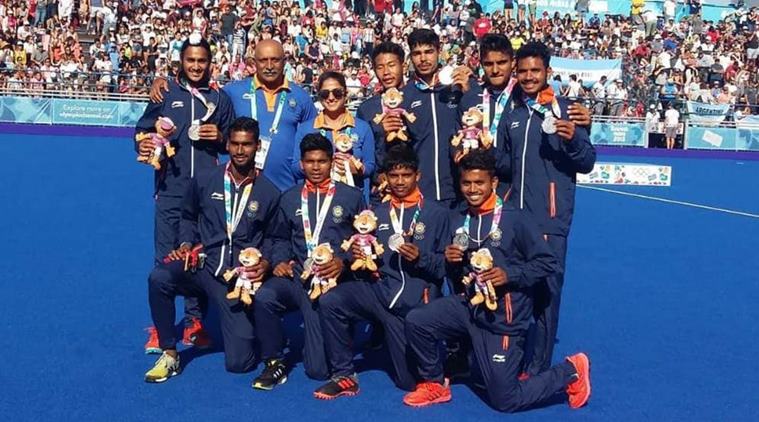In this vibrant outdoor photograph, a triumphant team of athletes is captured celebrating their competition victory in broad daylight. The wide horizontal image showcases a dark blue court, bordered by a blue barrier separating the athletes from a densely packed crowd of spectators in ascending stands. The audience, some holding signs and flags, adds to the jubilation of the scene. 

The team, predominantly comprised of men of Indian or Southeast Asian descent, is attired in dark blue jumpsuits, each proudly displaying a silver medal around their necks. The athletes are also holding small stuffed toys, reminiscent of tiger figures. In the back row, seven men stand tall, while the front row features four men kneeling. Notably, the second person from the left in the standing row appears to be the coach, distinguished by his gray mustache and light blue shirt, with another woman in a similar outfit beside him. The unified stance and beaming expressions of the team encapsulate their shared moment of glory.